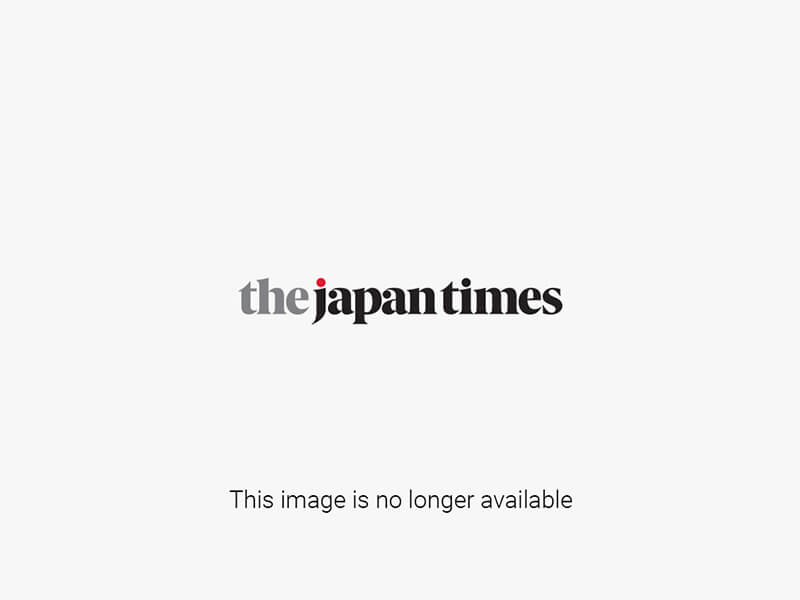The image captures a detailed action shot of an Asian male baseball player in mid-pitch, his left leg lifted high in the air. The focus is sharp on him, revealing his expression of intense effort with his mouth open, while the background is a muted blur, likely a stadium crowd, textured in whites and grays. He wears a black baseball cap with a red letter, a white pinstriped jersey with black stripes, and the word "JAPAN" along with the number 16 on the front. His undergarment is a long-sleeve, black New Balance shirt. He completes his outfit with matching pinstriped pants and gray shoes with red laces. His hair is dark black, his eyes are dark, and he lacks any facial hair, conveying a clean and focused athlete in peak condition. His left fist is clenched around a mitt, indicative of his pitching motion.